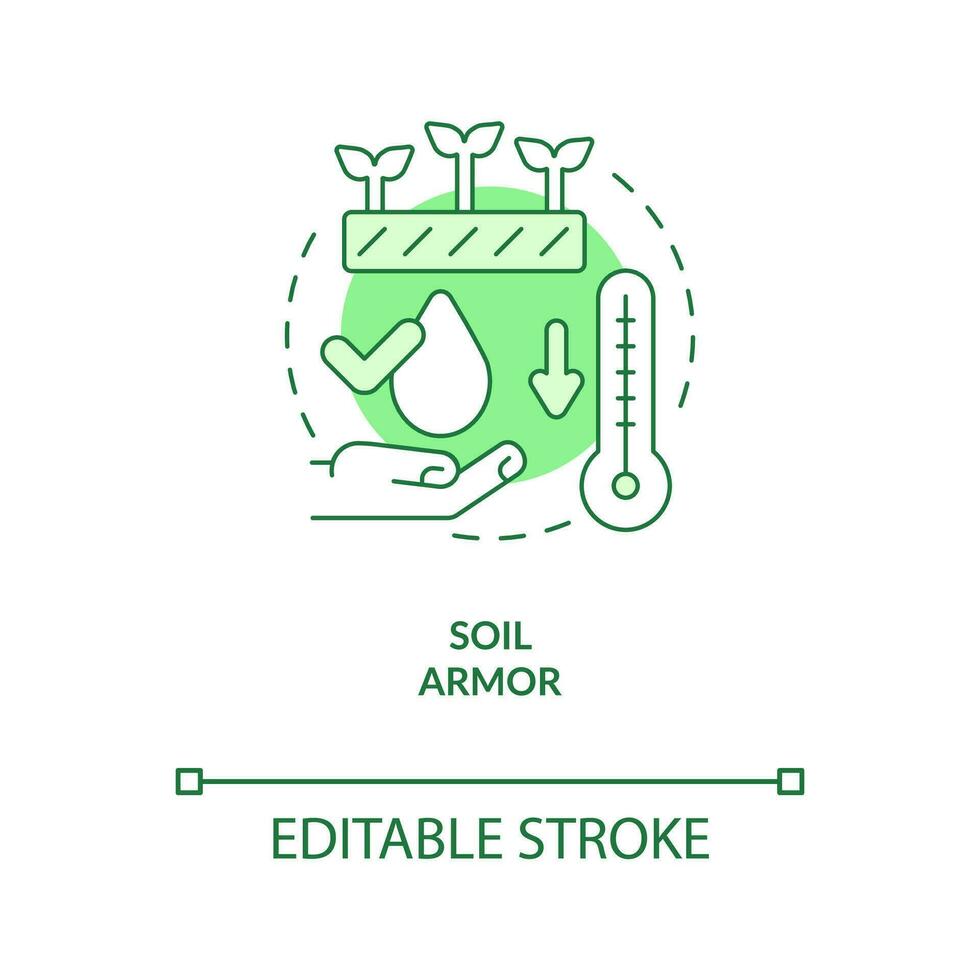The image features a white background with several green elements and text. Starting at the bottom, the words "Editable Stroke" are written in green letters. Above this phrase, there is a horizontal line with small squares at each end. Directly above this line, the phrase "Soil Armor" is also displayed in green. Encircling this text is a dotted green line forming a broken circle. Within the circle, several green symbols are arranged: a box with lines and a two-leaf stem sprouting from it (repeated three times), a checkmark, a teardrop symbolizing water, an arrow pointing downward, a thermometer, and a side view of a hand showing only the thumb and index finger extended. At the center of the circle is a shaded green circle.